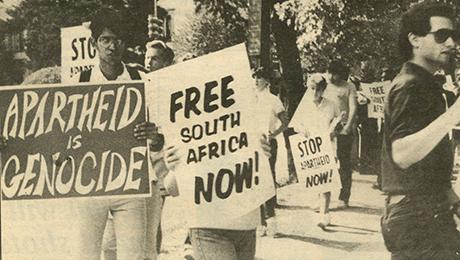This black-and-white photograph, likely taken between the 1950s and 1970s, depicts a protest against apartheid in South Africa. The image captures a diverse group of young people, including men and women, marching along a road lined with trees. The protesters hold up various signs with powerful messages: "Apartheid is Genocide," "Free South Africa Now," and "Stop Apartheid Now." Among the marchers, one individual on the right stands out, wearing glasses and a short-sleeved shirt tucked into jeans, while another appears on the far left. The demonstration scene evokes a significant historical struggle against the racist policies of apartheid in South Africa, reflecting the intense desire for freedom and justice during that era.